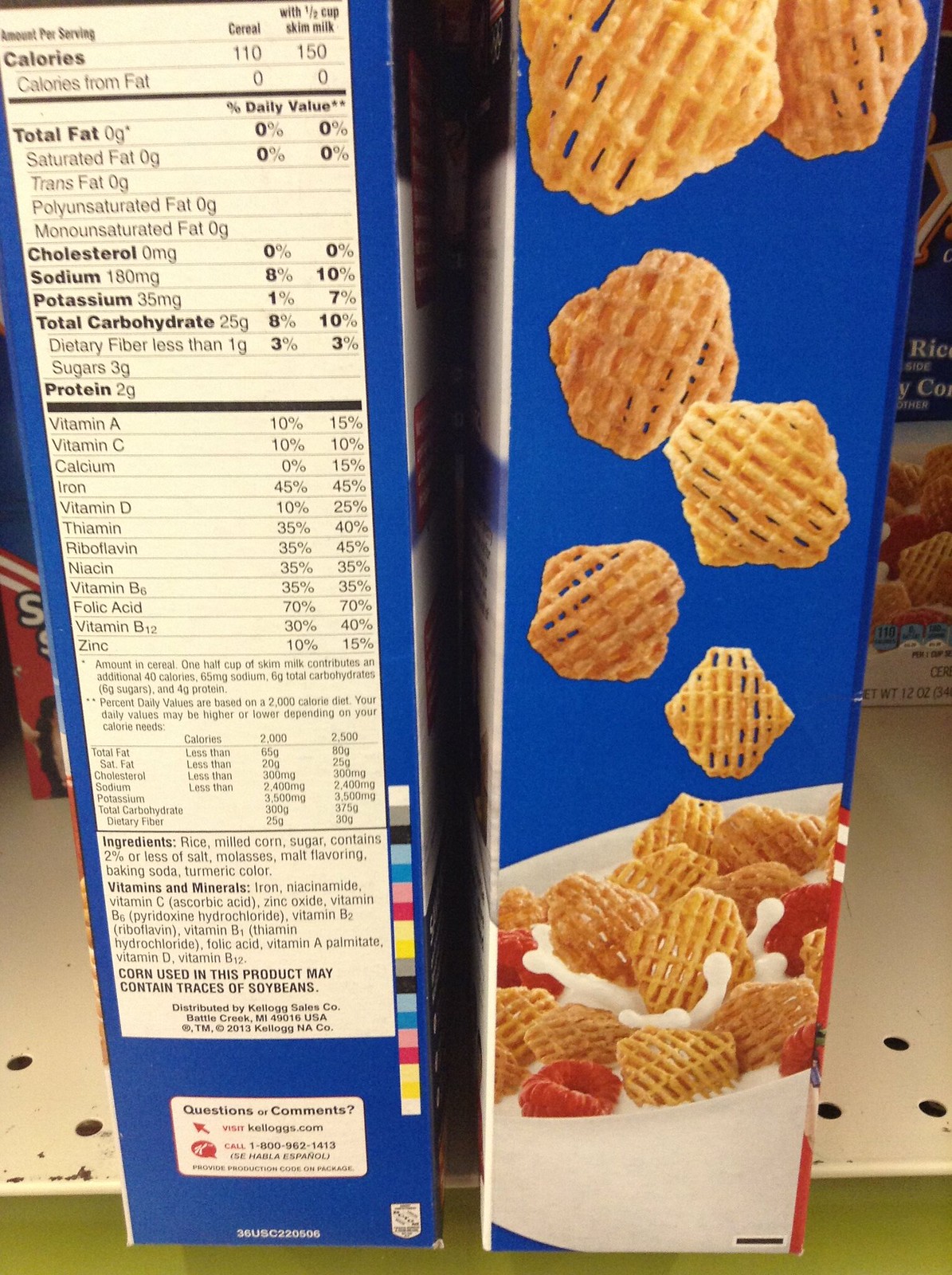This detailed photograph captures two side-by-side cereal boxes on a store shelf, viewed from the side panel. The left box prominently features a close-up image of the cereal, which resembles Rice Chex. The right box displays extensive nutritional information, detailing the calories, fat content, cholesterol, sodium, potassium, total carbohydrates, protein, and an array of vitamins and minerals. The ingredients list reveals that corn is used in the product and indicates the possibility of trace amounts of soybeans. As a Kellogg's product, it is likely either Corn Chex or Rice Chex. The packaging provides contact information for Kellogg's, including their website, kelloggs.com, and a 1-800 customer service number, which confirms bilingual support in English and Spanish.